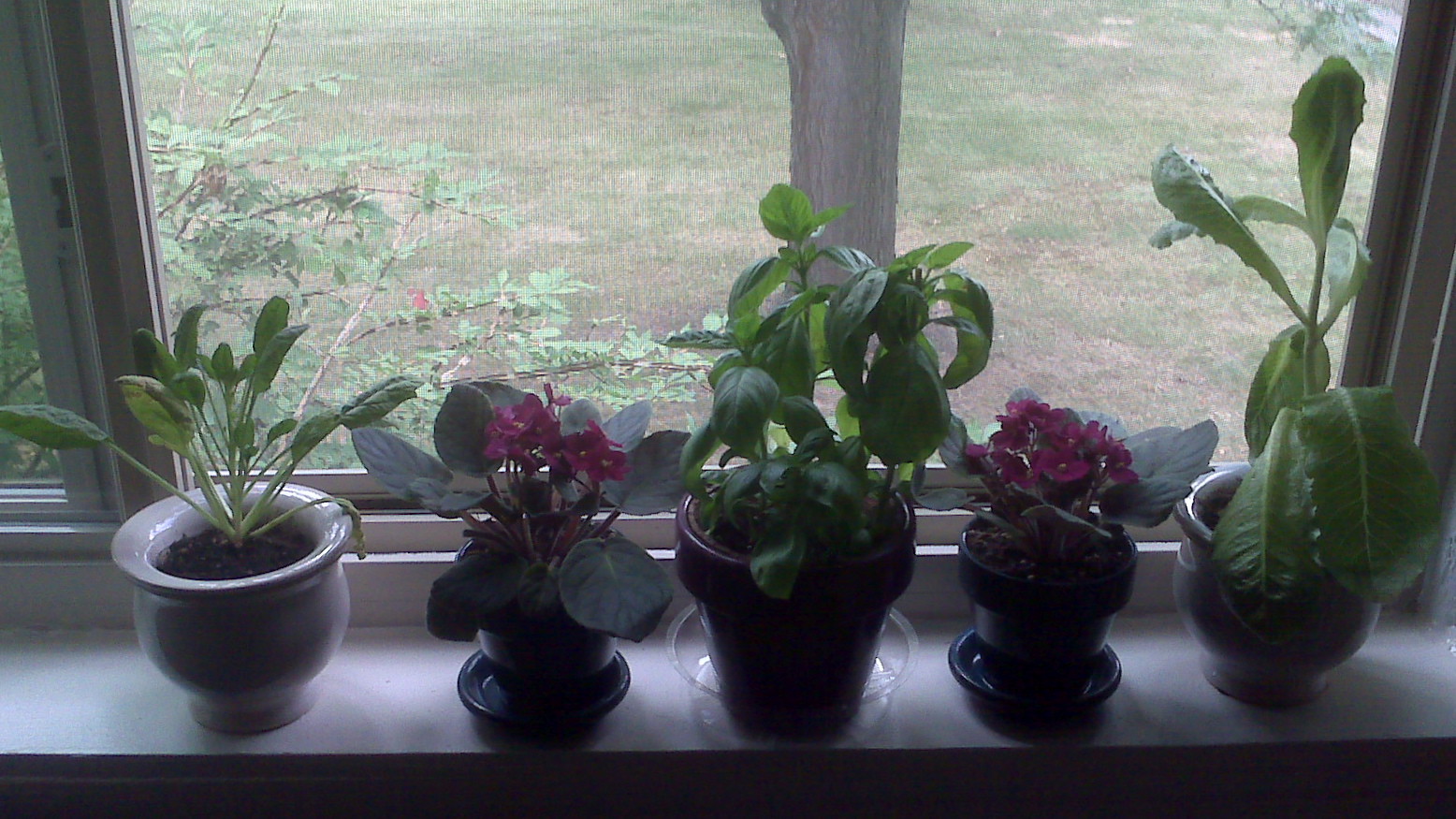This photograph captures the sunlit window of a residence, showcasing an array of five potted plants arranged on a white windowsill. The central focus is a lush basil plant situated in a dark brown or black ceramic pot, flanked by vibrant violet-colored flowers with dark green leaves in pots. Among these, the pot on the far left is distinctly white, while the pot on the far right is either white or light gray, obscured slightly by the dim lighting of an overcast day. Outside the open window with a visible screen, you can glimpse a yard with patchy, partially dying grass interspersed with green patches, along with a small tree and bush. The overall scene highlights the care taken to ensure the indoor plants receive ample sunlight, set against the serene and slightly melancholic backdrop of an overcast day.